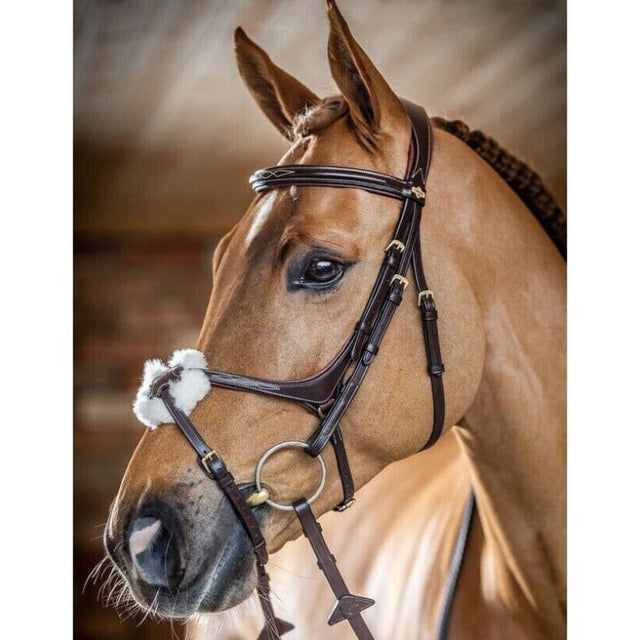This detailed photograph captures a close-up of a horse's head, predominantly showing the left side as the horse slightly turns its face to the right. The background is entirely out of focus, presenting a blurry brown shade that complements the horse's own brown coat. The setting suggests a structure with wooden elements visible at the top and in the backdrop, enhancing the earthy tones of the image. 

The horse's body can be vaguely seen in the background, contributing to the blurred effect, while the image sharply focuses on the intricate details of its face. The horse's head is adorned with a dark brown leather halter, meticulously stitched with golden thread and featuring gold brackets and emblems, adding a touch of elegance to the scene. 

Significantly, the horse has a distinctive white line running down the center of her forehead to between her eyes, with further touches of white on her nostrils and a lighter brown shading under her chin. Her nose and muzzle exhibit a blend of dark gray with speckles of black, contrasting her otherwise uniform brown coat. A protective, fluffy white cotton spacer is attached to the bridle around her nose, possibly to prevent irritation or provide comfort.

The horse has dark brown, expressive eyes highlighted by a black outline which adds depth to her gentle gaze. Her mane is neatly braided, contributing to her refined appearance. The overall composition emphasizes the blend of practical equestrian gear and the horse’s natural beauty in a softly muted background.